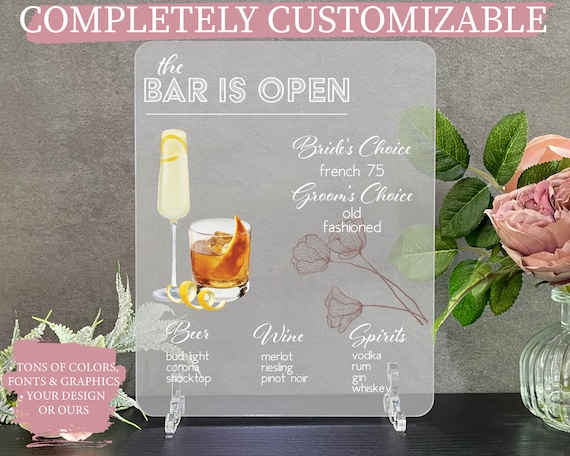This nearly square-shaped, horizontally oriented advertisement showcases a completely customizable product, likely from a company similar to Vistaprint or Canva. The bottom of the image features a dark, possibly cherry or black wood table, on which a frosted, partially transparent rectangular sign with clear legs stands. The sign reads "THE BAR IS OPEN" and depicts illustrations of a cocktail, as well as lists of various beers, wines, and spirits. Highlighted drinks include the Bride’s Choice, a French 75, and the Groom’s Choice, an Old Fashioned.

In the lower right corner of the image, part of a glass vase with pink flowers and green leaves is visible. The lower left corner displays an irregularly shaped pink background featuring bold white text that states, "TONS OF COLORS, FONTS AND GRAPHICS, YOUR DESIGN OR OURS." At the top, another pink background with white capital letters declares, "COMPLETELY CUSTOMIZABLE." This advertisement effectively illustrates the range of customizable design options available, from fonts and graphics to full templates for events such as weddings.